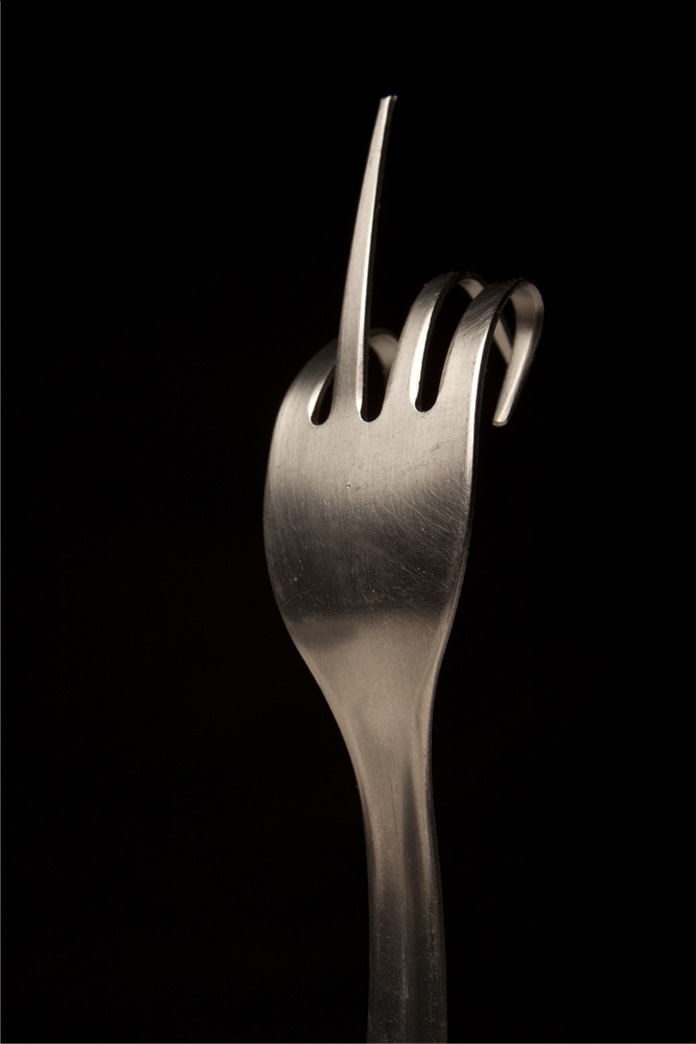The image is a close-up photograph of a shiny silver fork set against a completely black background. The visible portion of the handle extends only an inch or two from the bottom of the frame before it fades into the blackness. The focus is on the tines of the fork: the leftmost tine and the two rightmost tines are all bent sharply forward, almost folding back into the lower half of each tine. The second tine from the left, however, stands straight up as it normally would. This unusual bending gives the appearance that the fork is making a crude gesture, reminiscent of giving a middle finger. The silver surface of the fork reflects light in varying degrees of brightness, adding a subtle glint against the dark backdrop.